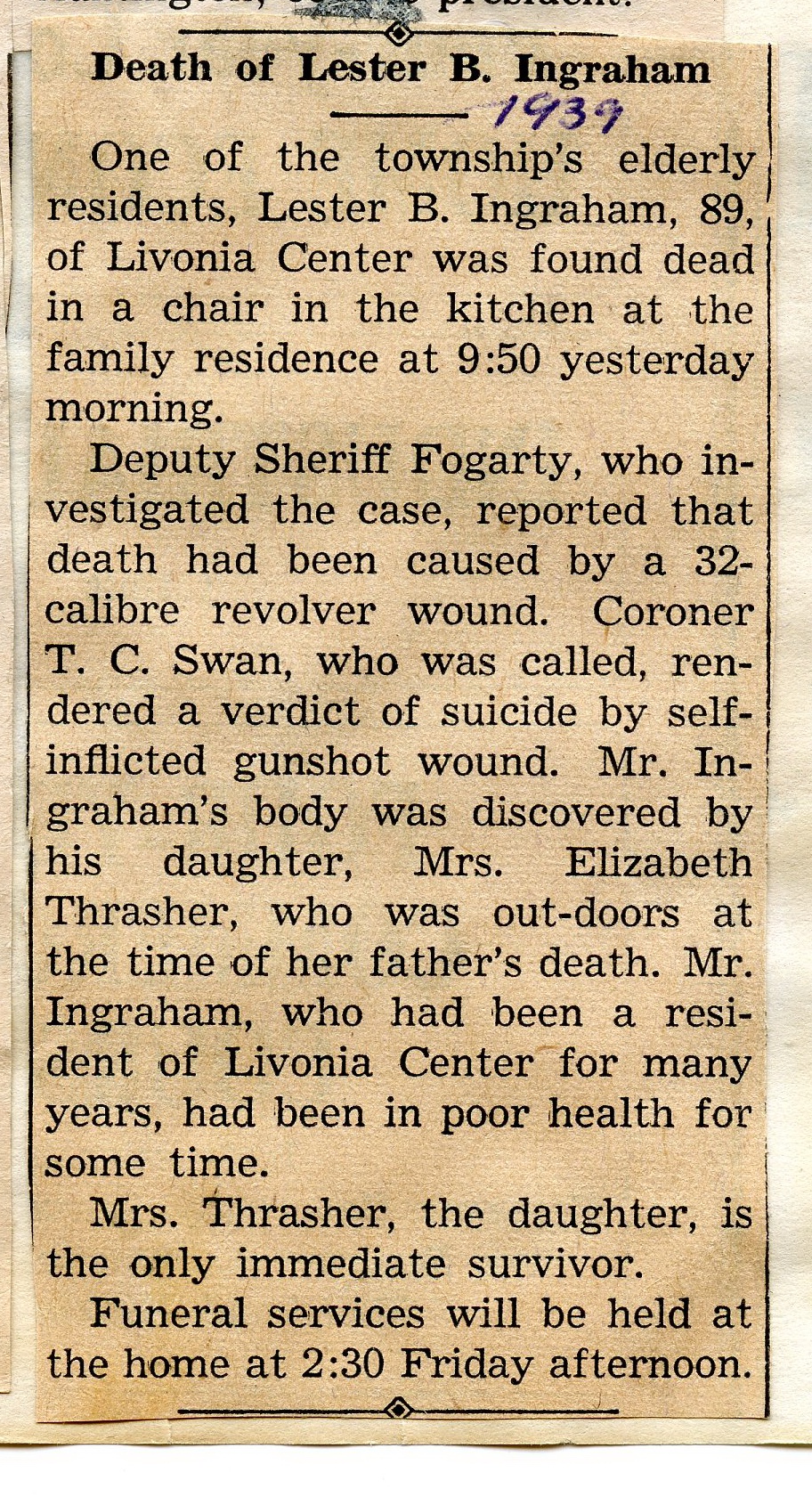The image is a photograph of a newspaper clipping that appears to be scanned. The paper has a beige, aged look with black text and a handwritten note in blue ballpoint pen that reads “1939” under the headline. The headline states, "Death of Lester B. Ingraham." The article details the death of one of the township's elderly residents, Lester B. Ingraham, aged 89, of Livonia Center. He was found dead in a chair in the kitchen at the family residence at 950 yesterday morning. Deputy Sheriff Fogarty, who investigated the case, reported that death was caused by a .32 caliber revolver wound. Coroner T.C. Swan rendered a verdict of suicide by self-inflicted gunshot wound. Mr. Ingraham's body was discovered by his daughter, Mrs. Elizabeth Thrasher, who was outdoors at the time of her father's death. Mr. Ingraham, who had been a resident of Livonia Center for many years, had been in poor health for some time. Mrs. Thrasher is the only immediate survivor. Funeral services are scheduled to be held at the home at 2:30 PM on Friday afternoon.